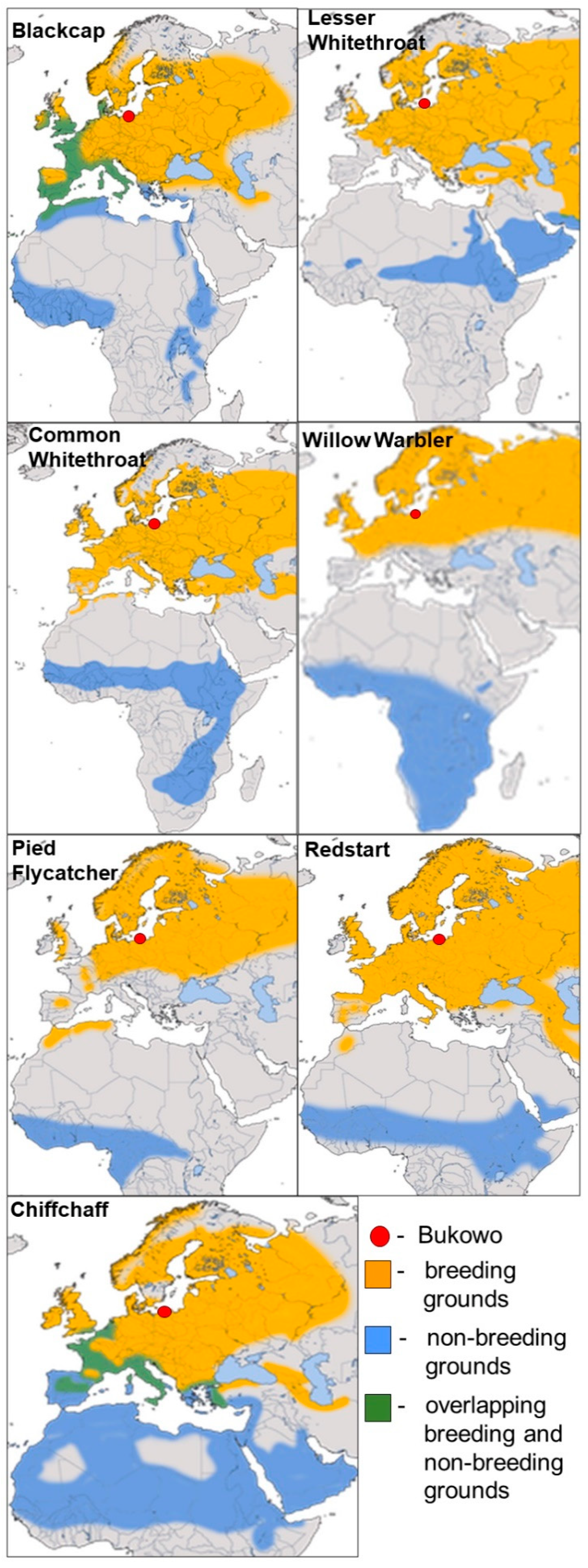This digital chart displays geolocational data, mapping the breeding, non-breeding, and overlapping grounds of various bird species across multiple continents, specifically Europe and Africa. The chart is segmented into seven detailed maps, each labeled with the names of bird species: Black Cap, Lesser Whitethroat, Common Whitethroat, Willow Warbler, Pied Flycatcher, Redstart, and Chiffchaff. 

Each map features color-coded regions—yellow for breeding grounds, blue for non-breeding grounds, and green for overlapping regions. In addition, each map has a distinct red dot, marked with "Bukowo," highlighting a specific area. The top left map, labeled "Black Cap," shows notable colored regions in both Europe and Africa, while subsequent maps, such as "Lesser Whitethroat" and "Common Whitethroat," continue to highlight areas within Europe. The legend in the bottom right corner aids in interpreting these color codes and geographical markers. The chart serves as a comprehensive visual representation of the habitats and migratory patterns of these bird species.